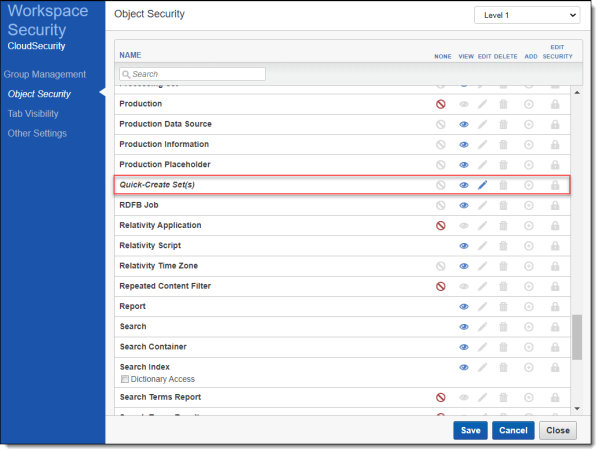This image is a detailed screen capture of a user interface related to workspace security and object management settings. 

To the left side of the image, a blue column lists navigation options in white text. The headings include "Workspace Security" and "White Cloud Security," followed by sections for "Group Management," "Object Security," indicated by a white arrow, "Tab Visibility," and "Other Settings."

On the right side, the image displays a white background populated with black text, interspersed with blue text elements. At the top, it reads "Object Security Level 1," next to a pull-down menu labeled "Name" highlighted in blue. The menu options include "None," "View," "Edit," "Delete," "Add," and "Edit Security." Below this, there is a white search box for easy navigation.

Further down, a series of black text listings are visible, each with associated icons indicating levels of access or functionality. For example:
- "Production" has a red circle next to it.
- "Production Data Source" is marked with a blue eye icon, indicating visibility.
- "Production Information," "Production Placeholder," and "Quick Create Sets" each have a blue eye, with "Quick Create Sets" also featuring a blue pencil, indicating edit permissions.
- "RDFB Job" is marked with a blue eye.
- "Relativity Application" and "Relativity Script" both have red circles.
- "Relativity Time Zone" and "Repeated Content Filter" feature a blue eye and a red circle, respectively.

Following, several items—"Report," "Search," "Search Container," and "Search Index"—all have a blue eye icon. There is a white box labeled "Directory Access" adjacent to these items. Further down, "Search Terms Report" exhibits a red circle. The list continues with additional entries partially cut-off, still marked with red circles.

At the bottom of the screen, the interface features three action buttons: a blue "Save" button and a "Cancel" button, both with white text, and a gray "Close" button with black text.